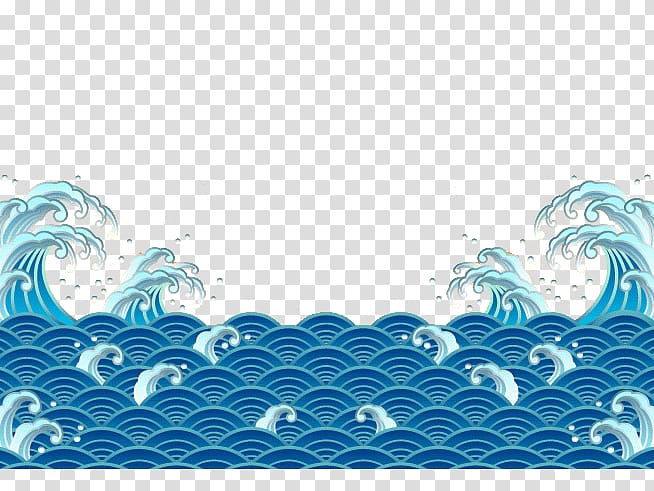This detailed, cartoon-like vector illustration portrays a stylized section of a body of water. The entire composition is symmetrical, with each side mirroring the other exactly. The main elements are the waves, predominantly depicted with upward arcs resembling segments of concentric circles, creating a geometric, scale-like effect. The waves transition from dark blue at their base to light blue at the edges, lending depth and contrast to the image. Some waves rise higher and curl into spheres, rendered in lighter shades of blue and white, adding dynamic movement. Larger waves are positioned towards the outer edges of the artwork, with medium-sized waves more centrally located. Behind the waves is a gray and white checkerboard pattern, indicating transparency for easy removal, ensuring the waves remain the focal point. This artistic choice enhances the overall clean and defined visual style characteristic of vector drawings.